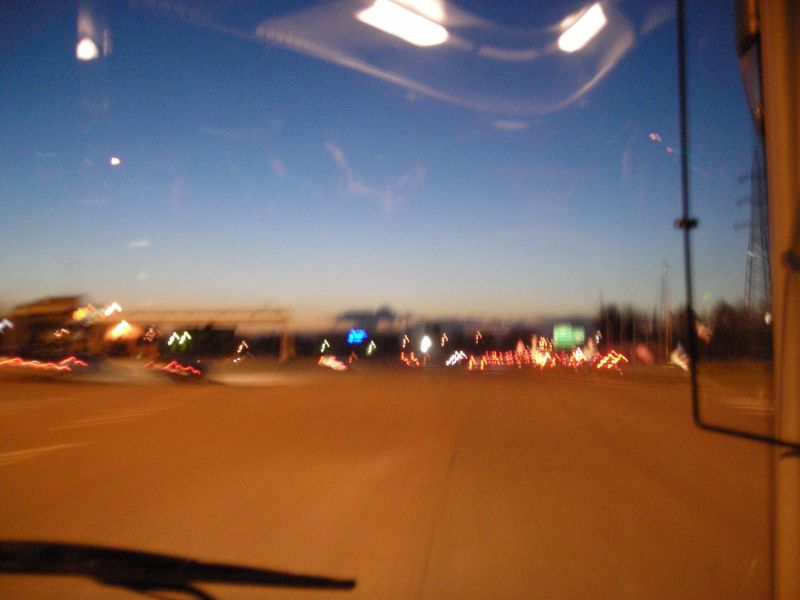The photograph captures a scene from inside a bus, looking out through the windshield onto a bustling freeway. It was taken during the early evening, as the sky is transitioning from day to dusk. The setting sun casts a dimming light, making the scene gradually darker. In the distance, numerous cars with their brake lights illuminated create a red haze, indicating a possible traffic slowdown.

To the left side of the image, a large overhead sign towers over the freeway, providing guidance to drivers. Below it, the silhouette of a building can be seen, adding to the cityscape. On the right side of the frame, clusters of trees are visible, interspersed with a prominent power pole that cuts vertically through the scene. The blue sky above begins to show signs of twilight, while a slight blur encompasses the brake lights and distant cars, suggesting motion and the bus's forward journey.